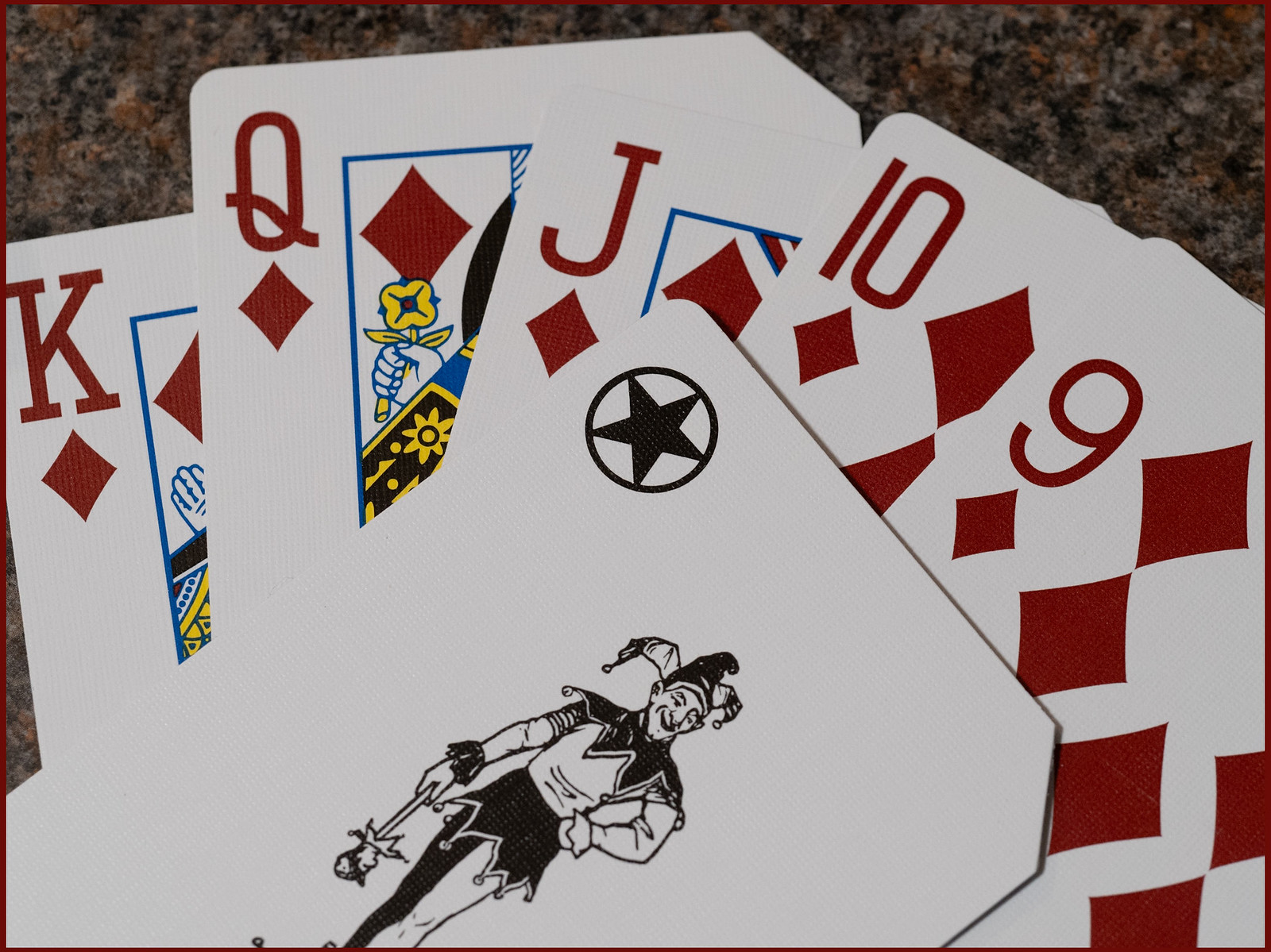Against a predominantly black background with speckles of gray and black, there is a stand of playing cards extending from the left to the right. On the left side of the stand, the sequence of cards includes the Queen, King, Jack, Ten, and Nine of Diamonds. In the forefront, there's a prominently displayed Joker card. 

The Joker card features intricate details: at the top left corner, there's a circle enclosing a black star. The central figure on the card, the Joker, wears a traditional jester hat and displays a cheerful smile. The Joker's right hand is placed on his hip, while his left hand holds a staff adorned with a head at the end, folded downwards. His costume includes a neckline decorated with triangular patterns, and he wears a black skirt paired with mismatched stockings—one white and one black. 

Surrounding the Joker are multiple thin lines, adding complexity to the background of the card. Notably, the top right corner of the card appears to be flat. The Queen of Diamonds card, located on the left side, features a yellow flower, and there's a rectangle on this card adorned with a yellow flower pattern as well.